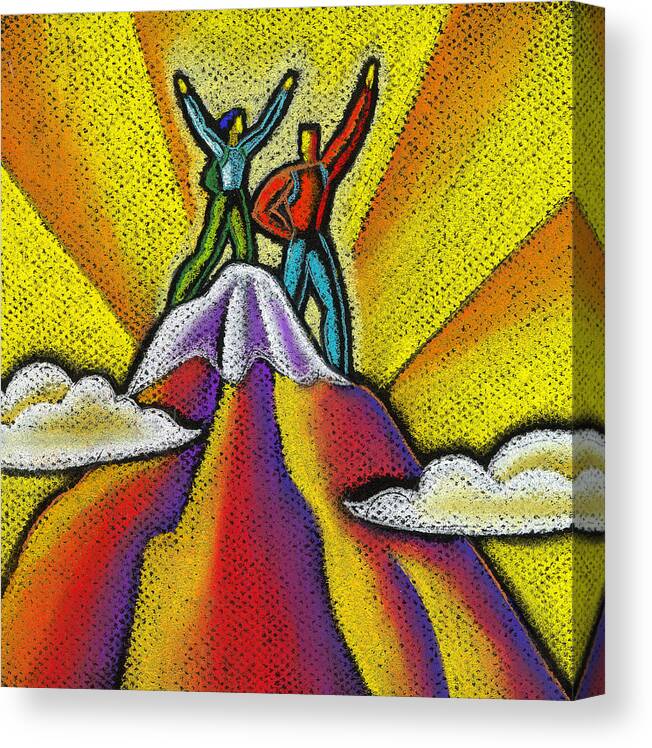This vibrant and whimsical painting on canvas depicts a cartoonish scene of a man and a woman celebrating their triumph at the summit of a colorful mountain. Bathed in the warm hues of an orange and yellow sky, the setting sun radiates behind them, adding a sense of achievement to the moment. The mountain beneath their feet is a kaleidoscope of purples, reds, and yellows, and its snow-capped peak sits just above the fluffy clouds. The man, dressed in a long-sleeve red shirt and blue jeans, extends his left arm in a victorious gesture while his right arm is poised behind his back. A backpack is slung over his shoulders, suggesting a challenging ascent. Beside him, the woman exudes joy, with both arms raised high. She is clad in a long-sleeve blue shirt, green pants, a green backpack, and a blue hat. Their jubilant stance captures the exhilarating accomplishment of reaching the top of the mountain.